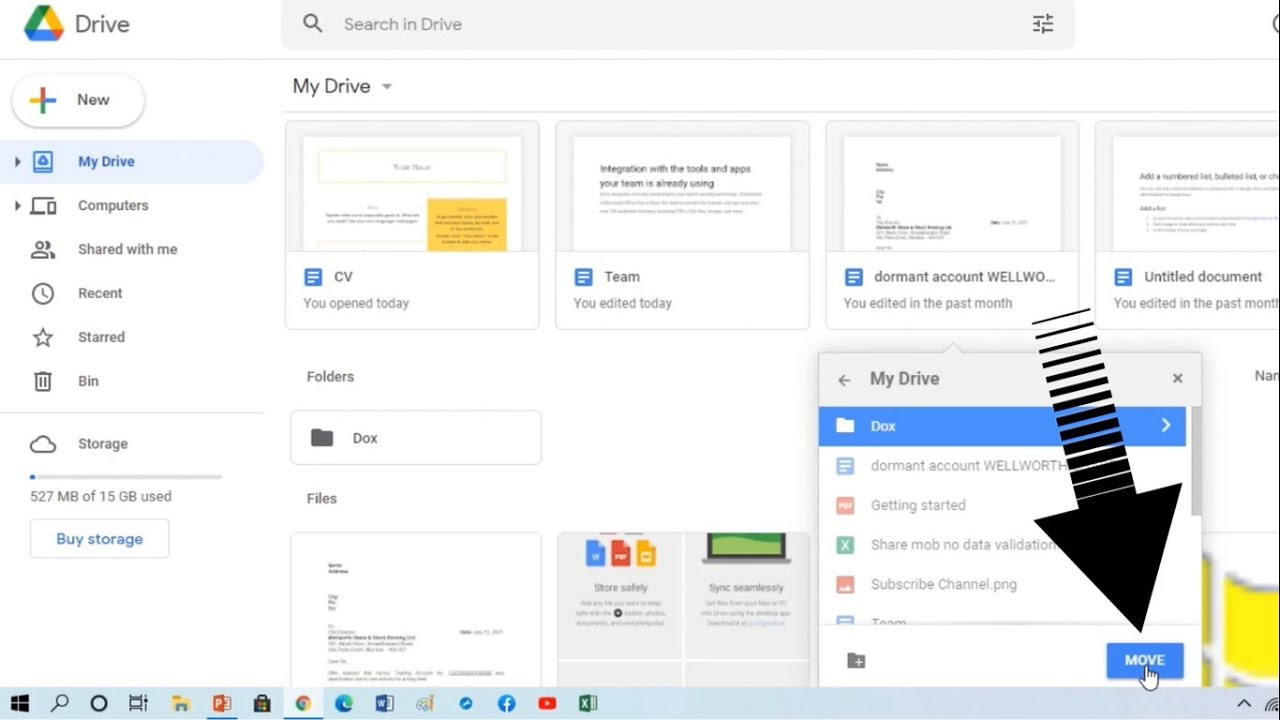The image is a screenshot of the Google Drive home page, specifically the 'My Drive' section, as indicated by the highlighted blue color on the left side of the screen. The left panel also includes various categories such as Computers, Shared with Me, Recent, Starred, and Bin, with Storage appearing further down. In the Storage section, there is a status bar displaying "527 MB of 15 GB used," accompanied by a "Buy Storage" button beneath it. On the bottom right side of the screenshot, there is a prominent black arrow pointing downward towards a blue button labeled "Move," which appears to be located within a separate pop-up box or function window.